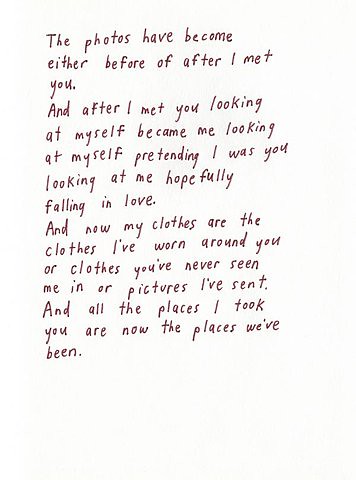The image shows a piece of paper with a subtle light gray, almost pinkish background, and features three paragraphs of handwritten text in brown ink or marker. The text reads: "The photos have become either before or after I met you. And after I met you, looking at myself became me looking at myself, pretending I was you, looking at me, hopefully falling in love. And now my clothes are the clothes I've worn around you, or clothes you've never seen me in, or pictures I've sent. And all the places I took you are now the places we've been." The handwriting is neatly left-aligned, giving the impression of a personal, perhaps obsessive, love letter or poem.